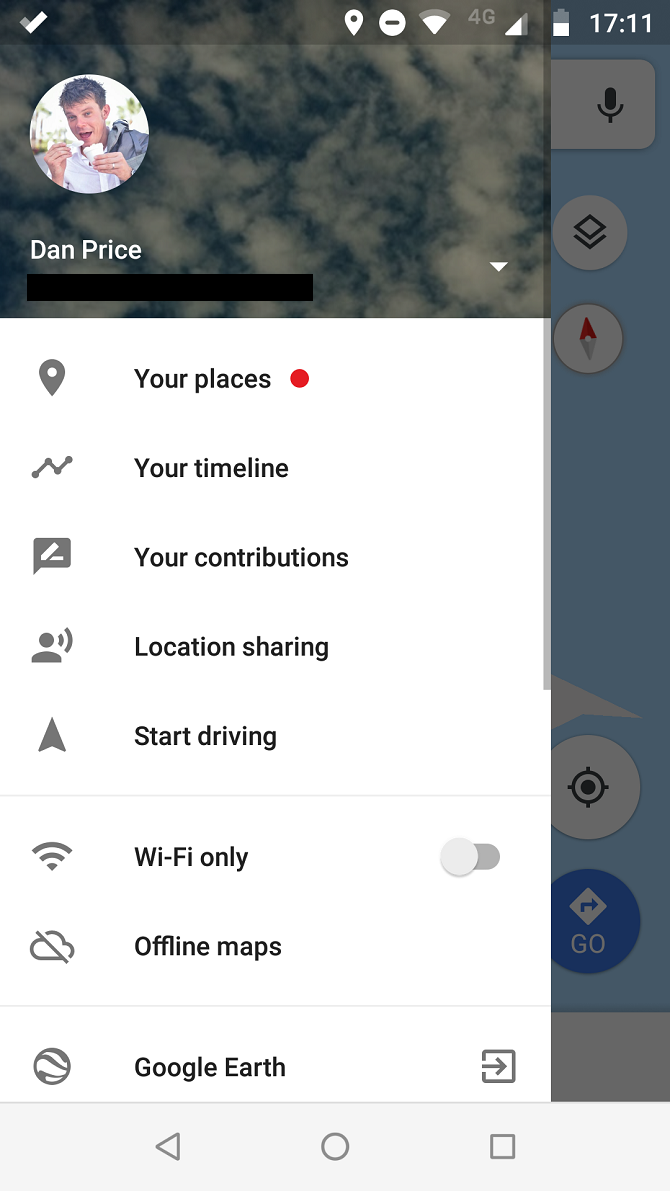Screenshot of a smartphone taken in portrait orientation, captured at 17:11, with approximately half battery life remaining and a 4G connection with moderate signal strength. The GPS is active, displaying Google Maps. The screen shows a profile selection menu for "Dan Price," depicted as a young white male, likely in his teens or twenties, holding a cup of yogurt or a similar item in his left hand. The profile picture is prominently featured at the top left. Below the profile picture, several menu options are listed: "Your places" (for frequently visited or important locations), "Your timeline" (a history of visited locations), "Your contributions" (likely user reviews or photos), "Location sharing" (sharing real-time location with others), "Start driving" (navigation mode), an unticked "Wi-Fi only" mode, "Offline maps" (for map access without an internet connection), and "Google Earth" (for satellite and 3D views).